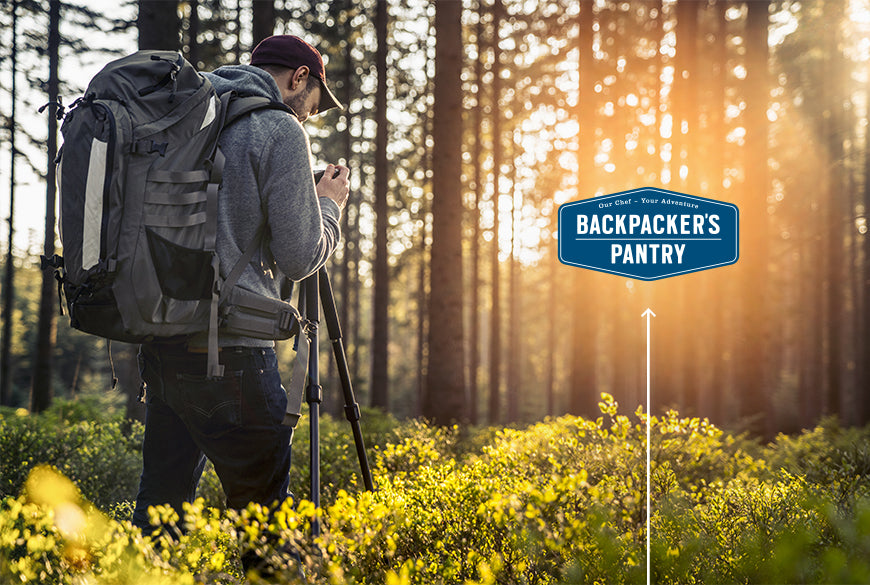In this digitally generated advertisement set in a daylight forest scene, vibrant greenery and tall trees are illuminated by sunlight streaming through sparse leaves. Dominating the right-hand side of the image is a prominent blue sign with a white arrow pointing toward it. The sign, hexagon-shaped with white borders, bears the slogan "Our Chef, Your Adventure" and the brand name "Backpackers Pantry." 

To the left stands a bearded man, seen from the back, who is deeply engaged with his camera equipment. Dressed in a gray hoodie, dark blue jeans, and a maroon baseball cap, he steadies a digital camera on a tripod with his right hand. A large, gray backpack, possibly by Backpackers Pantry, is slung over his shoulders, emphasizing the adventure theme of the scene. The lush, light green plants at ground level and the bright, sunlit background enhance the outdoor appeal of the image, suggesting an exciting exploration into the wilderness.